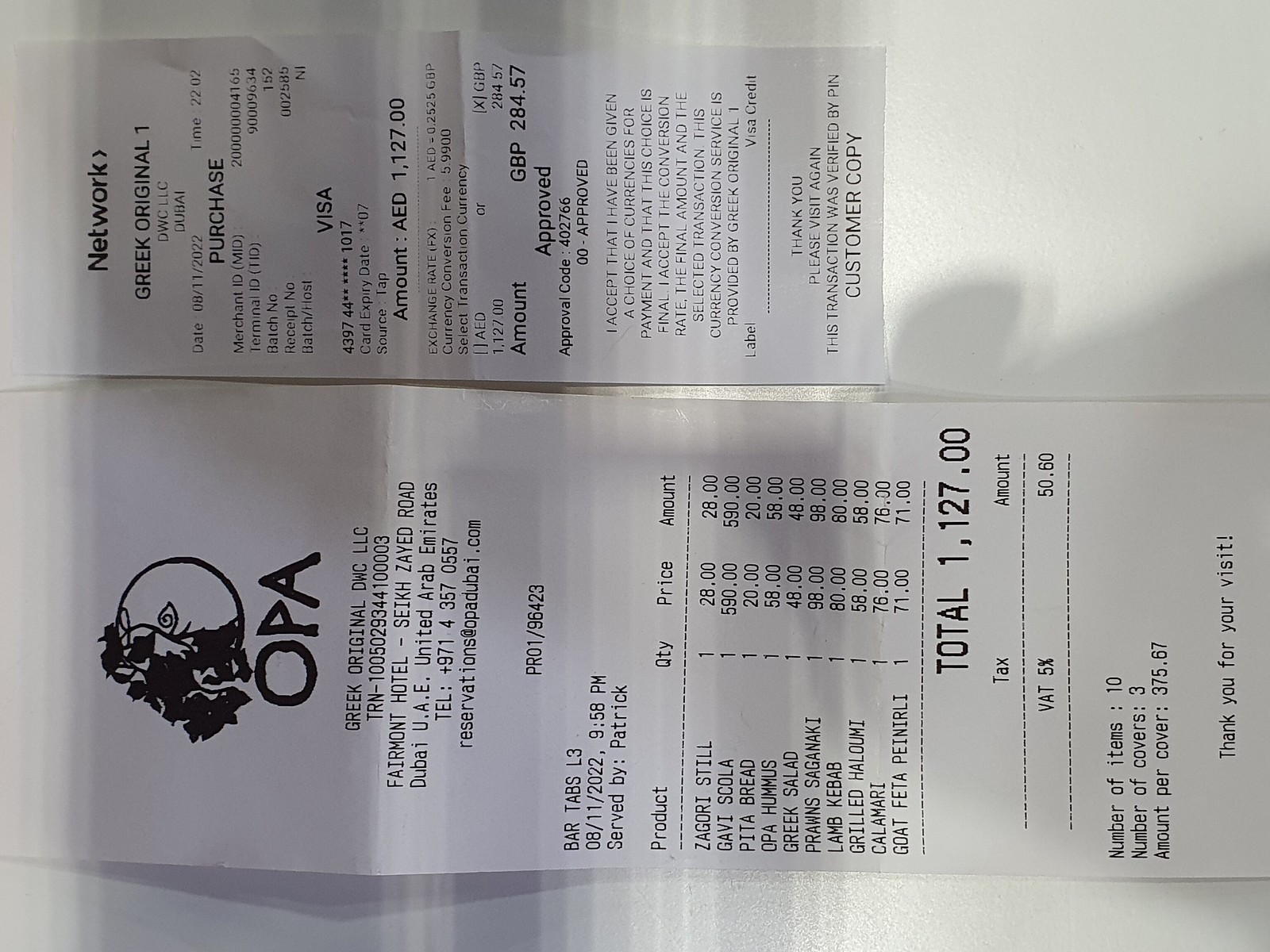In the image, there are two receipts positioned horizontally, side by side. The top receipt is from the establishment "Network," and it appears to be shorter in length. The bottom receipt, significantly longer, is from "OPA," which is identified as either a Greek restaurant or a Greek food shop. The total amount paid on the OPA receipt is £1,127. Both receipts include a VAT rate of 5%. The receipts might also pertain to card payments and possibly include an additional tipping service fee. The arrangement and detail of the receipts suggest a careful comparison or analysis of recent expenditures at these establishments.